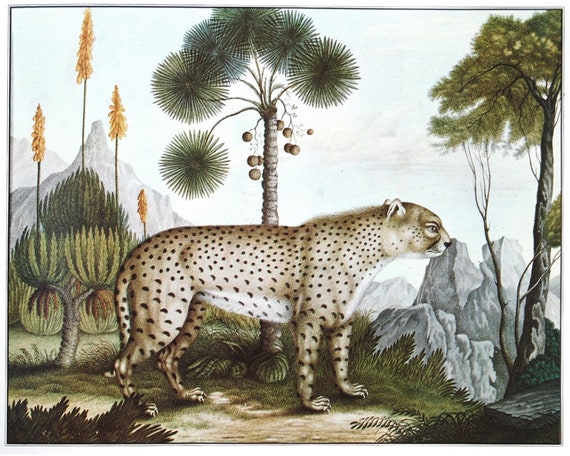This is a stylized painting featuring a leopard-like big cat standing in the center on a brown dirt path, with a white belly and pale beige fur adorned with black spots. The feline's body is presented in full profile, facing right, with its tail hanging to the left. The head is dark brown on top, fading to light brown underneath, with a black nose and white around the mouth. Short, white ears sit atop its head. Surrounding this central figure, the scene includes various elements of tropical nature. Directly behind the cat stands a distinctive tree with gray trunks, often described as resembling palm or Joshua trees, featuring dark green, starburst-like leaves and clusters resembling coconuts or fruit. To its left is a shorter tree with light green, pointy leaves, and behind it to the right, a tall tree with a crown-shaped top and yellowish-green leaves. More into the distance on the left, there are extraordinarily tall, thin brown trunks topped with golden smudges. The background is further enriched by exaggerated gray mountains and a pale blue sky. The painting combines realistic elements with a slightly flat, illustrative quality, perhaps reminiscent of colonial or vintage styles.